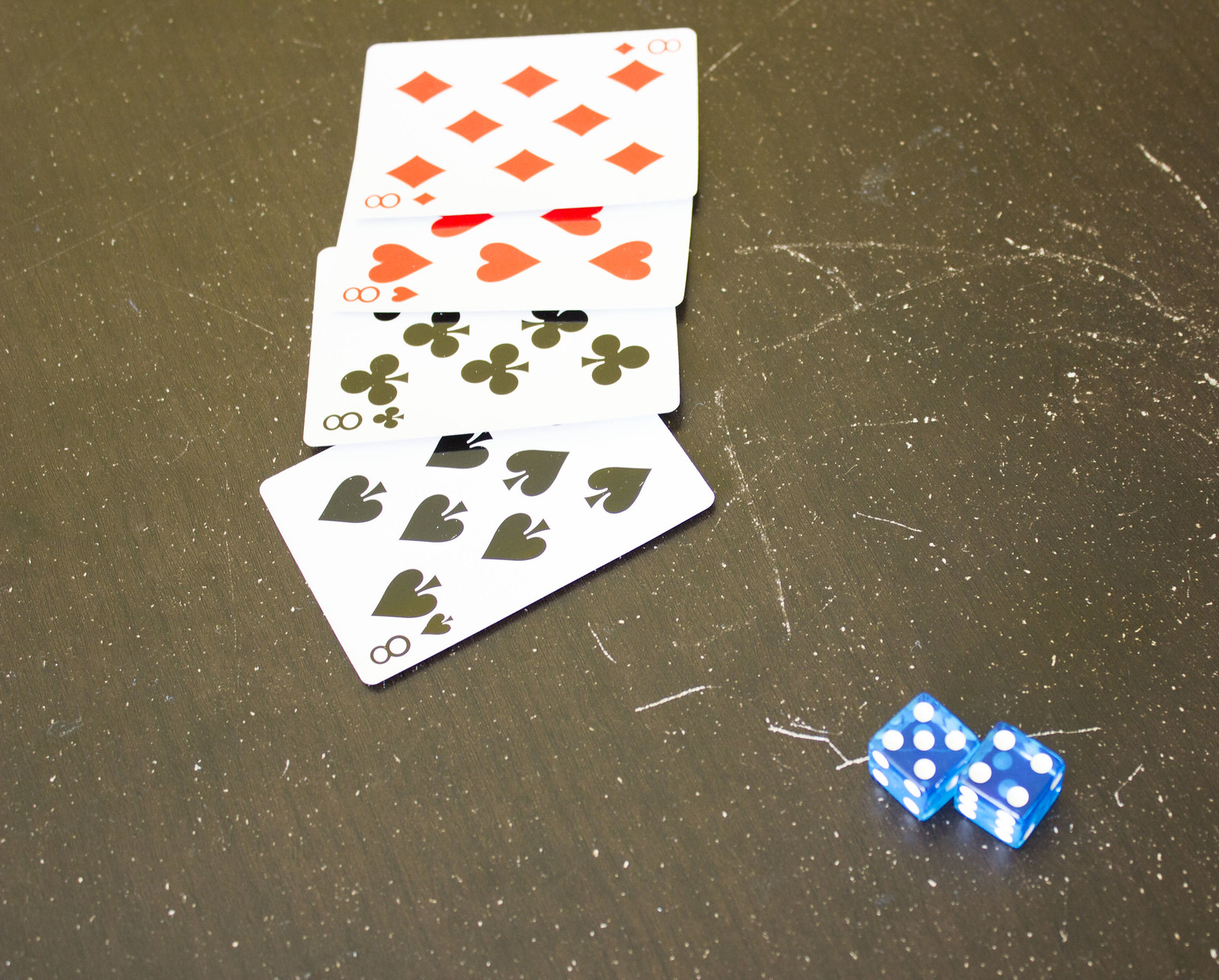An old, heavily worn, brown table, its surface marred by deep scratches, nicks, and numerous paint flecks revealing years of use, serves as the backdrop. Atop the table, two blue dice with white dots are shown, displaying a roll of five and four. Amongst them lie four playing cards neatly arranged: the eight of clubs, eight of spades, eight of hearts, and eight of diamonds, suggesting a remarkably good hand. The juxtaposition of the dice and cards hints at a game in progress, though its nature remains unclear. The table's rustic, chipped paint and rough, uneven texture tell a story of countless games and gatherings over time.